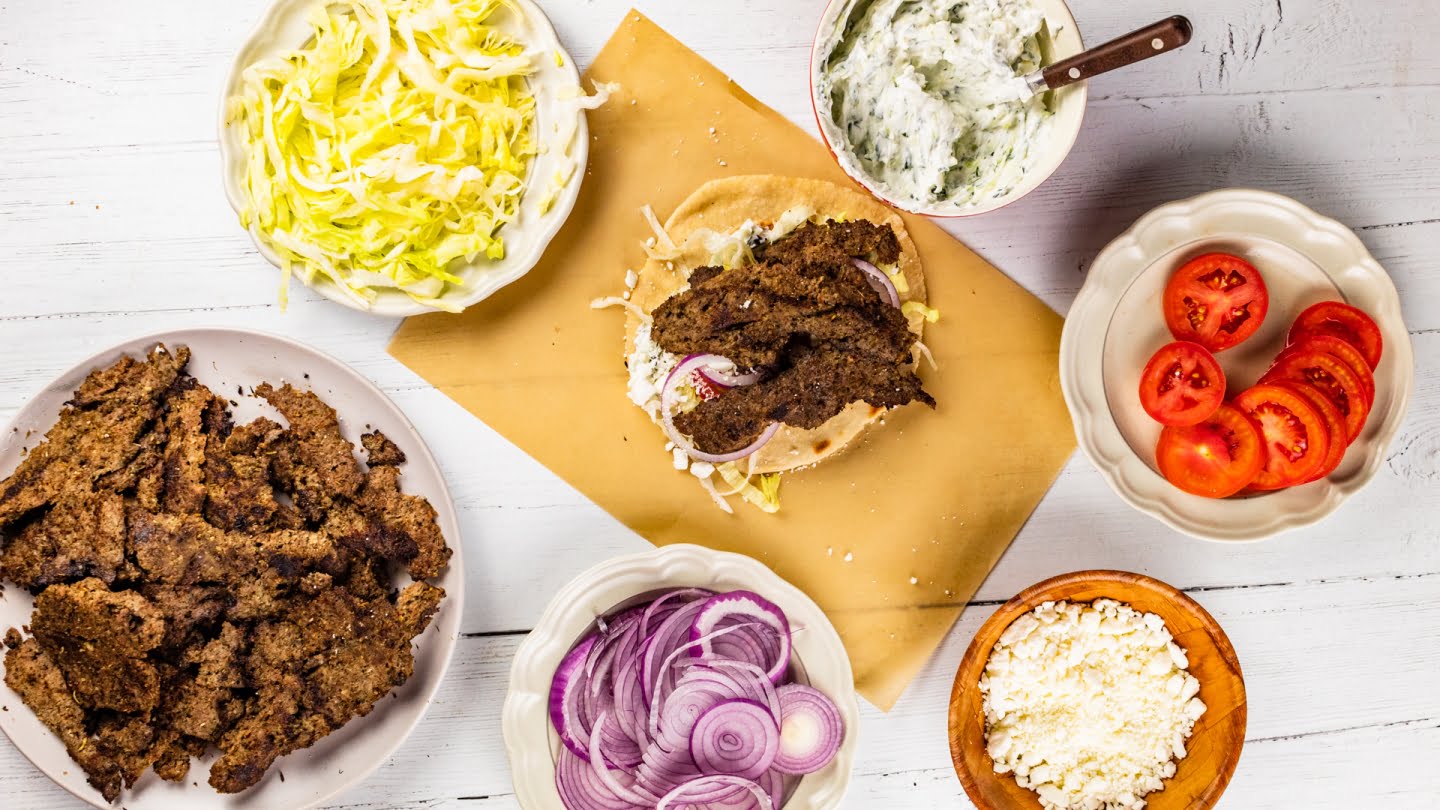The image depicts a top-down view of a light wooden table painted white, adorned with an assortment of seven assorted plates and bowls filled with various ingredients spread out neatly. Central to the arrangement is a piece of brown parchment paper topped with a tortilla. On the tortilla rests a mix of fresh lettuce, both red and regular onions, and a portion of browned, grilled meat, suggestive of a burrito in the making. Directly to the right is a white dish containing neatly arranged tomato slices. Below this, a wooden bowl holds a quantity of crumbled cheese. Adjacent to it, a white bowl contains diced red onion. To the left of the parchment paper, a white plate displays additional grilled meat. Another white plate nearby is filled with shredded lettuce strands. Finally, a bowl with a thick white sauce speckled with herbs, is positioned with a wooden spoon sticking out of it, ready for serving. The compilation of these ingredients creates an inviting scene best suited for a publication on recipes or culinary presentations.